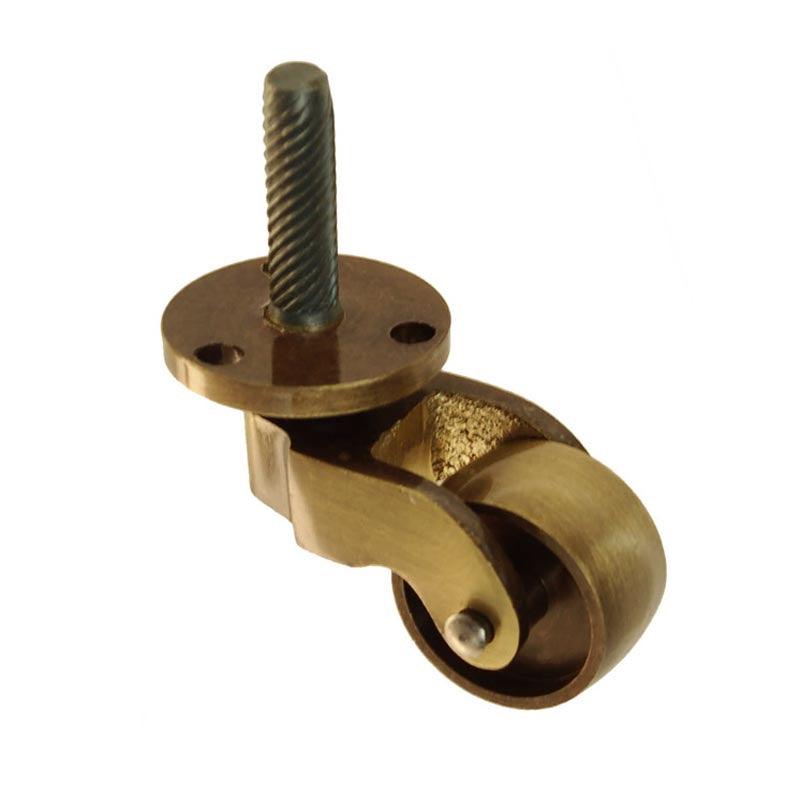This detailed product photo showcases a brass antique caster designed for furniture. The caster wheel is entirely made of metal, displaying a worn brass finish indicative of its vintage nature. The wheel is housed in a brass holder, anchored by a fastener that secures the wheel to the housing. The attachment mechanism features a distinct threaded fastener meant for a precise application, likely involving the installation into a drilled hole in wood. Below the wheel, there is a round base plate with multiple screw holes for additional stability when affixed to furniture. The image appears meticulously edited or photographed against a plain white background to emphasize the product’s details, highlighting its heavy-quality brass construction and robust design.